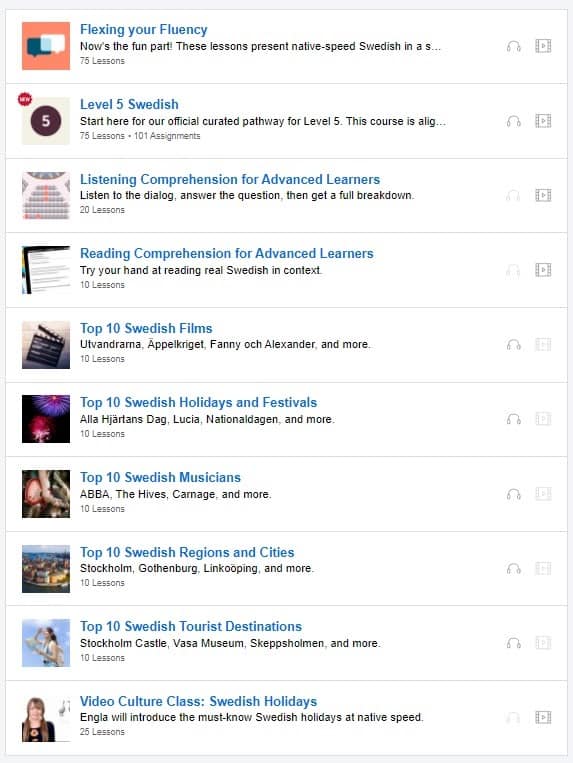Here is a well-structured, detailed caption for the screenshot of the website:

---

This screenshot captures an educational website, likely a language learning platform, displaying an extensive list of courses and classes designed to teach Swedish. The courses are organized in a comprehensive column format, each featuring a distinct title and description.

1. **Flexing Your Fluency**: Highlighted in blue font, this course offers an immersive experience with native-speed Swedish. Learners can delve into a total of 75 lessons to enhance their fluency.

2. **Level 5 Swedish**: This course is the official curated pathway for advanced learners at Level 5, consisting of 75 lessons and 101 assignments, providing a structured and thorough curriculum for serious language enthusiasts.

3. **Listening Comprehension for Advanced Learners**: Aimed at honing advanced listening skills, this course includes 20 lessons where students listen to dialogues, respond to questions, and receive detailed breakdowns.

4. **Reading Comprehension for Advanced Learners**: This program challenges learners to read authentic Swedish text in context, comprising 10 intensive lessons focused on improving reading skills.

5. **Top 10 Swedish Films**: A cinematic journey through Swedish culture with movies like "Udvandorna," "Appelgurgit," and "Fanny Alexander." The course offers 10 lessons, each dedicated to a notable film.

6. **Top 10 Swedish Holidays and Festivals**: With 10 lessons, this course explores traditional Swedish celebrations such as Algeharterdag, Lucia, and Nationaldagen, among others.

7. **Top 10 Swedish Musicians**: Spanning 10 lessons, learners can discover prominent Swedish artists like ABBA, The Hives, and Carnage, blending language learning with musical influence.

8. **Top 10 Swedish Regions and Cities**: This course introduces learners to major Swedish regions and cities such as Stockholm, Gothenburg, and Linköping, across 10 detailed lessons.

9. **Top 10 Swedish Tourist Destinations**: Featuring iconic landmarks like Stockholm Castle, Vasa Museum, and Skeppsholmen, this 10-lesson course offers a virtual tour of Sweden’s top tourist spots.

10. **Video Culture Class: Swedish Holidays**: Led by Engla, this 25-lesson video series provides an in-depth introduction to essential Swedish holidays, narrated at native speed for authentic listening practice.

---

This caption provides a detailed and organized overview of the various Swedish courses available on the learning platform, making it clear and informative for users.